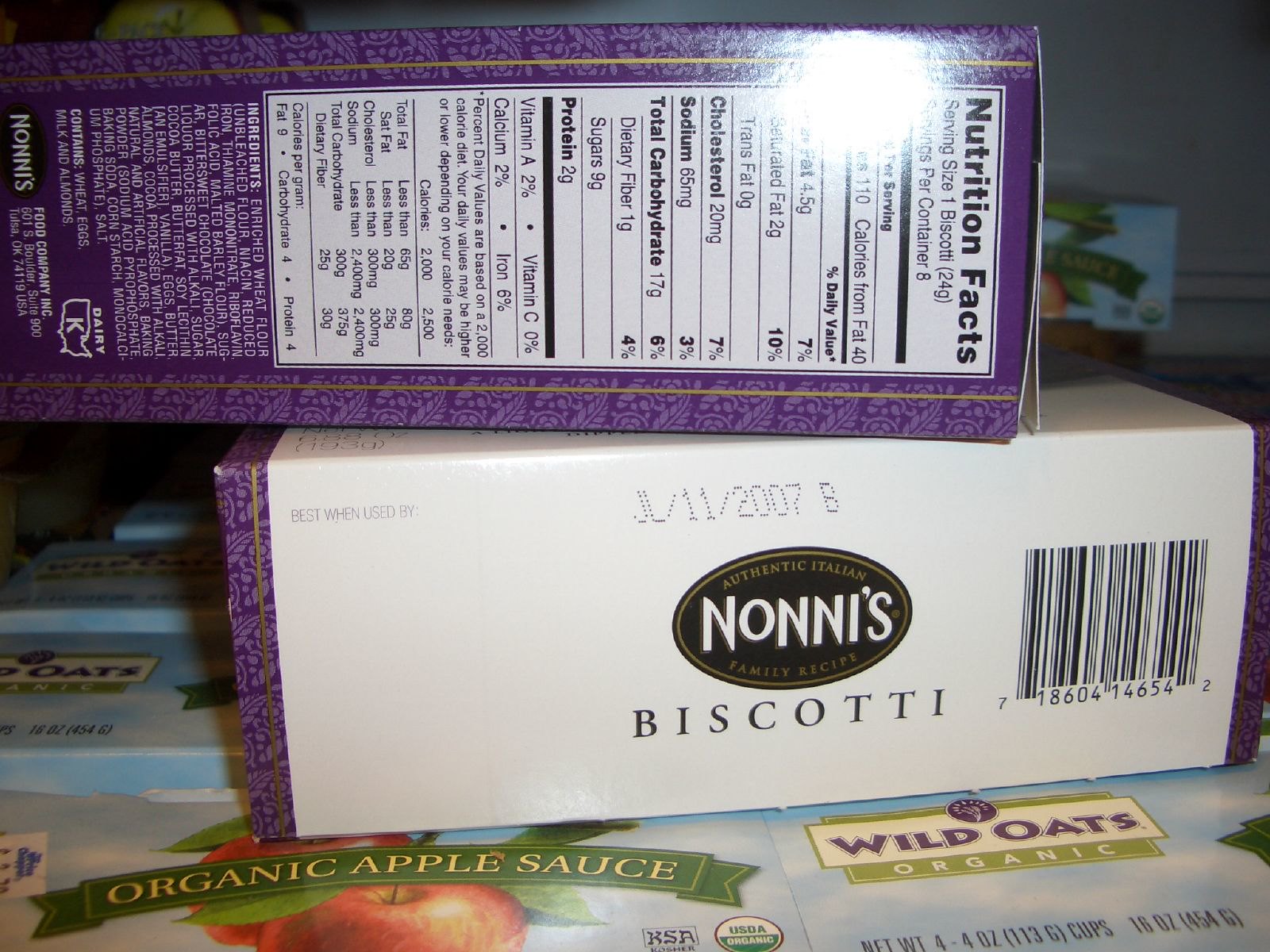The image features several stacked grocery items, seemingly placed either on a countertop, in a pantry, or inside a fridge. At the base, there's a box labeled "Wild Oats Organic," displaying the text "Organic Applesauce" alongside a picture of apples. This box indicates USDA Organic certification with a green and white emblem and details that it contains four 4-ounce cups, totaling 16 ounces. There's also a label in the lower right corner saying "Wild Oats Organic."

Placed directly on top of this applesauce box is a white box with purple edging on the left-hand side. This box prominently features the words "Authentic Italian Family Recipe" and "Nonni's" (spelled N-O-N-N-I-S) in a black oval, along with the word "Biscotti." Also visible are a barcode and an expiration date of July 11th, 2007.

At the very top of the stack is a primarily purple box, shown from the side to reveal a nutritional information label in a white rectangle. The label includes details such as serving size, and lists nutritional components like trans fats, cholesterol, sodium, total carbohydrates, protein, sugars, and dietary fiber in black text. This purple box appears to be another Nonni's biscotti box turned to display its side.